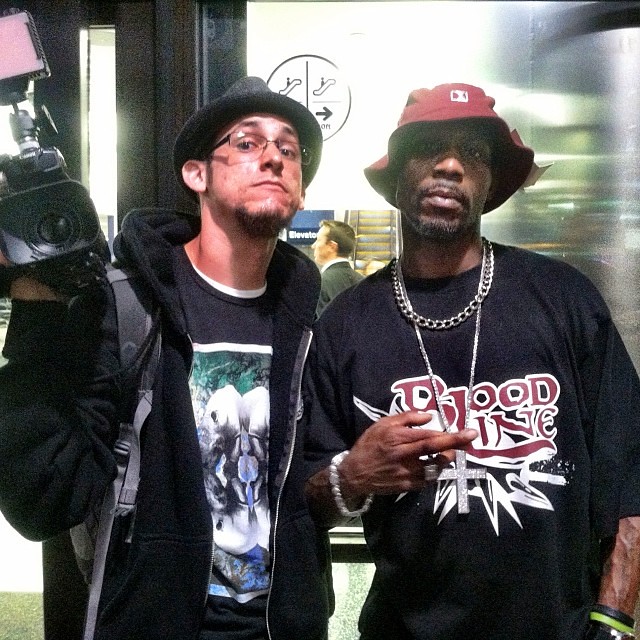In the vibrant image, two men stand prominently in the foreground, both facing the camera. On the left is a white man, recognizable by his goatee and glasses. He wears a gray hat, a black sweatshirt with a zipper down the middle, and a black t-shirt that seems to feature a colorful design in white, blue, and green. He holds a black camcorder in his right hand, resting it on his right shoulder. Straps, possibly from a bag, drape from his shoulder. On the right, a black man dons a striking red bucket-style hat. He sports a thick silver chain with a large silver cross, and his black t-shirt proudly displays the word "Bloodline" in bold red letters outlined in white. Both men have their chins slightly raised, exuding confidence. In the background, there's an escalator, gray and yellow, with a glimpse of a window above, and another person appearing between their heads. The setting suggests a busy, possibly public space, filled with dynamic elements and vivid colors.